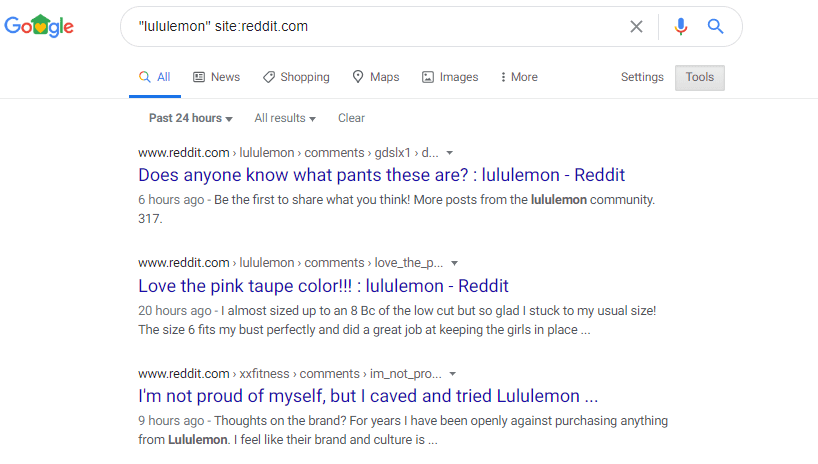A detailed screenshot taken on a desktop computer, displaying the Google search page. The screen features the prominent Google logo in the upper left corner. The search query entered is "lululemon" in quotation marks followed by "site:reddit.com," indicating an attempt to find information about Lululemon specifically from Reddit.com. Below the search bar, the various category buttons are visible, including All, News, Shopping, Maps, Images, More, Settings, and Tools. Additional filters include drop-down options for Past 24 Hours, All Results, and Clear.

The first search result is a Reddit post titled "Does anyone know what pants these are? – Lululemon Reddit." The second link is titled "Love the pink top color – Lululemon Reddit" with a partial description: “I almost sized up to an 8 because of the low cut but I'm glad I stuck to my usual size. The size 6 fits my bust perfectly and did a great job of keeping everything in place.” The third link reads, “I'm not proud of myself but I caved and tried Lululemon,” accompanied by a partial description: “Thoughts on the brand – for years I have been openly against purchasing anything from Lululemon. I feel like their brand and culture is...” The page has a white background with black text, and hyperlinks are displayed in blue.